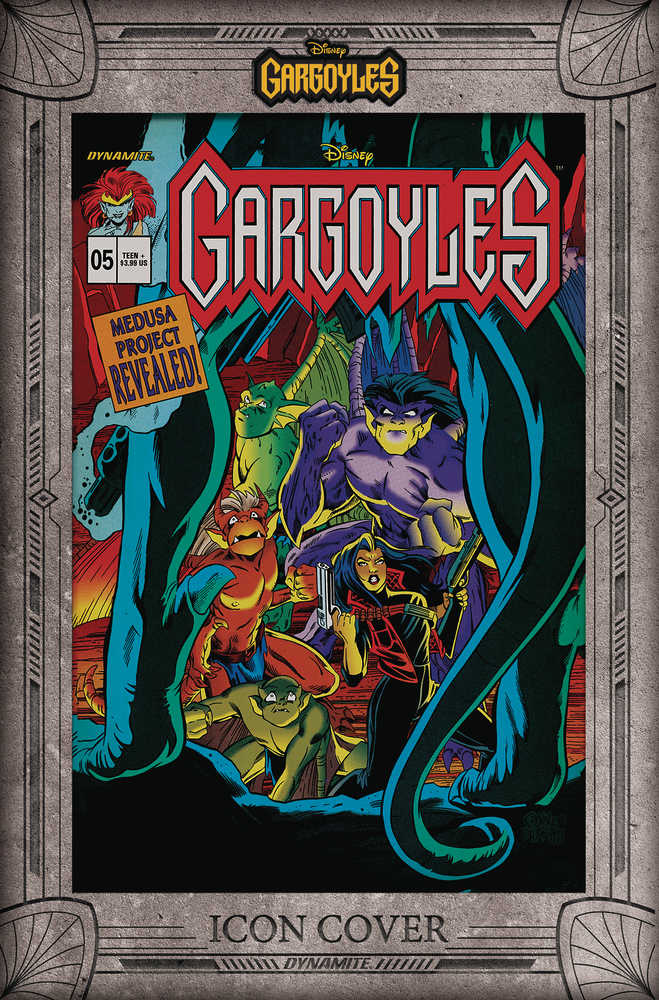The cover of a comic book titled "Disney's Gargoyles," likely a reprint of an iconic 90s issue, features a detailed and elaborate frame in a slate style with the text "Icon Cover Dynamite" at the bottom. Prominently, it showcases the diverse characters from the Gargoyles cartoon adaptation. Central to the cover is a human female with black hair, dressed in a red and black outfit, holding a gun. She is flanked by an array of gargoyle-like creatures: a green goblin-like creature crouching on all fours beneath her, a horned reddish creature standing beside her, and a muscular purple gargoyle with black hair towering above. All characters appear to be gazing intently at an unseen figure in the foreground, with only the demonic legs visible, reminiscent of traditional gargoyle statues. Additionally, a text box on the cover reads "Medusa Project Revealed," indicating a storyline within the comic.